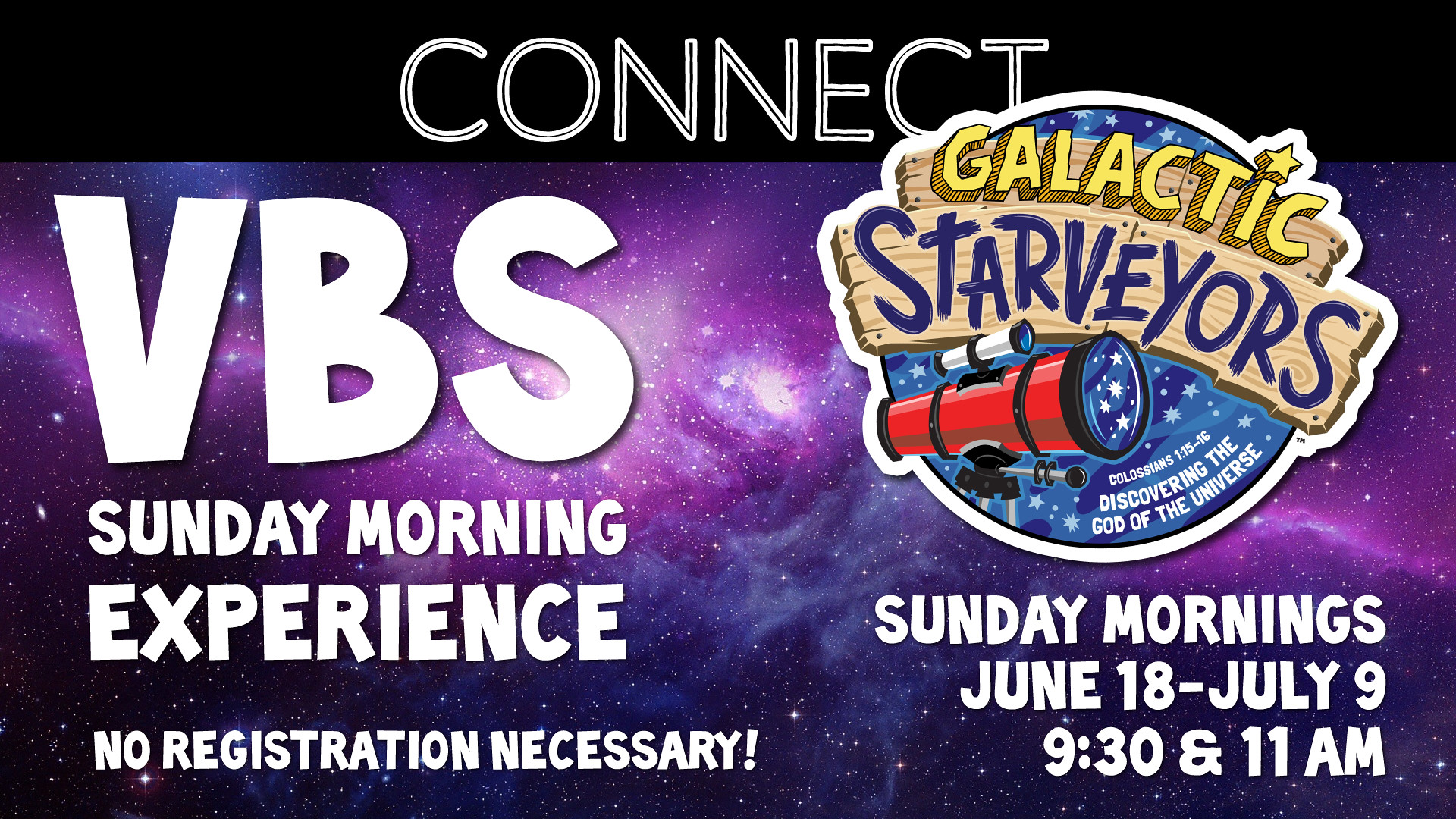The image is a detailed advertisement poster for a VBS (Vacation Bible School) Sunday morning experience. Dominating the top section, "Connect" is prominently displayed in white text over a black band that spans the width of the poster. Below this header, on the left, bold white text announces "VBS Sunday Morning Experience," emphasizing that "No Registration Necessary." To the right, under a wooden sign labeled "Galactic Starbears," there is an illustration of a telescope accompanied by the text "Discovering the God of the Universe," referencing Colossians 1:15-16. The event is scheduled for Sunday mornings from June 18th to July 9th, with sessions at 9:30 and 11:00 AM. The background is a vivid outer space theme, featuring a stunning purple and black galaxy adorned with bright stars and celestial imagery, creating a compelling visual that ties the whole advertisement together.